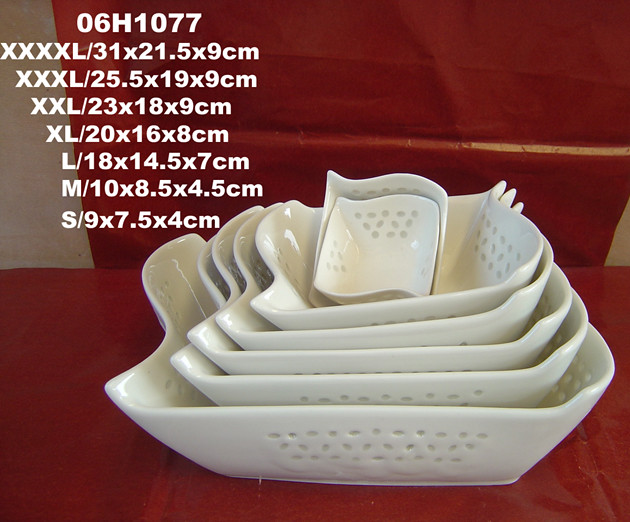The image portrays a set of seven ceramic or porcelain dishes, likely decorative or possibly strainers. The dishes are stacked within each other, with the largest at the bottom and each successive one smaller, presenting a nesting appearance. These dishes are primarily white and glossy, and they feature distinctive designs with holes or indentations on the sides. They are predominantly rectangular with dramatically wavy edges on the shorter sides, adding a unique flair to their shape. 

Two additional smaller square dishes, maintaining the same wavy design, can be seen nestled in the top dish. The entire arrangement sits on a shiny, red tablecloth, with another red fabric present in the background. In the upper left corner of the image, the text "06H1077" is visible, likely signifying a model number. To the right of this, the sizes are listed ranging from "XXXXL" to small, each accompanied by their respective dimensions.